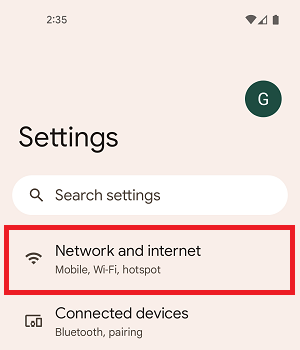This is a detailed screenshot of a smartphone's settings screen. The image appears to be cropped, omitting the phone's borders and other interface elements. The background is a subtle pinkish tan hue. The time displayed is 2:35. The smartphone shows full reception with a baseball diamond-shaped icon and the battery status icon is half full. A circular icon with a 'G' likely represents the user's initial or profile. 

At the top of the screen, there is a heading labeled "Settings" and a search bar with a magnifying glass icon, indicating a feature to search through the phone's settings. Below this, there is a section titled "Network & internet," which lists options such as "Mobile," "Wi-Fi," and "Hotspot." This section is distinctively highlighted with a red-bordered box, possibly for emphasis.

Further down, there's another section titled "Connected devices," which includes options like "Bluetooth" and "Pairing," accompanied by a relevant icon. Overall, the screenshot offers a concise view of the essential connectivity and device settings on the smartphone.